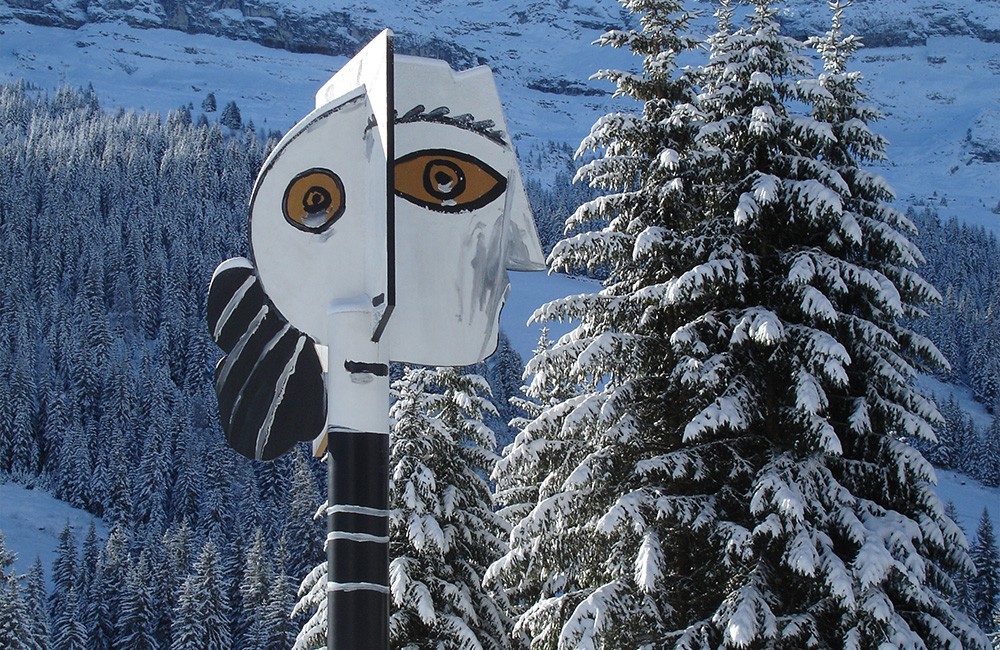This is a horizontally oriented photograph of a picturesque snowy forest scene, dominated by a collection of snow-covered evergreen trees. The foreground features several trees heavily laden with snow on their branches and needles, creating a pristine winter wonderland. To the left of the composition stands a striking black pole decorated with abstract, Picasso-esque art. This modern art piece features stylized faces with distinct yellow eyes, a triangular nose, and an eyebrow, reminiscent of Pablo Picasso’s surreal style. The sculpture's face profiles, one frontal and one side view, add an intriguing contrast to the natural setting. In the far background, above the tree line, snow-covered rocks are faintly visible, blending seamlessly into the idyllic winter landscape.